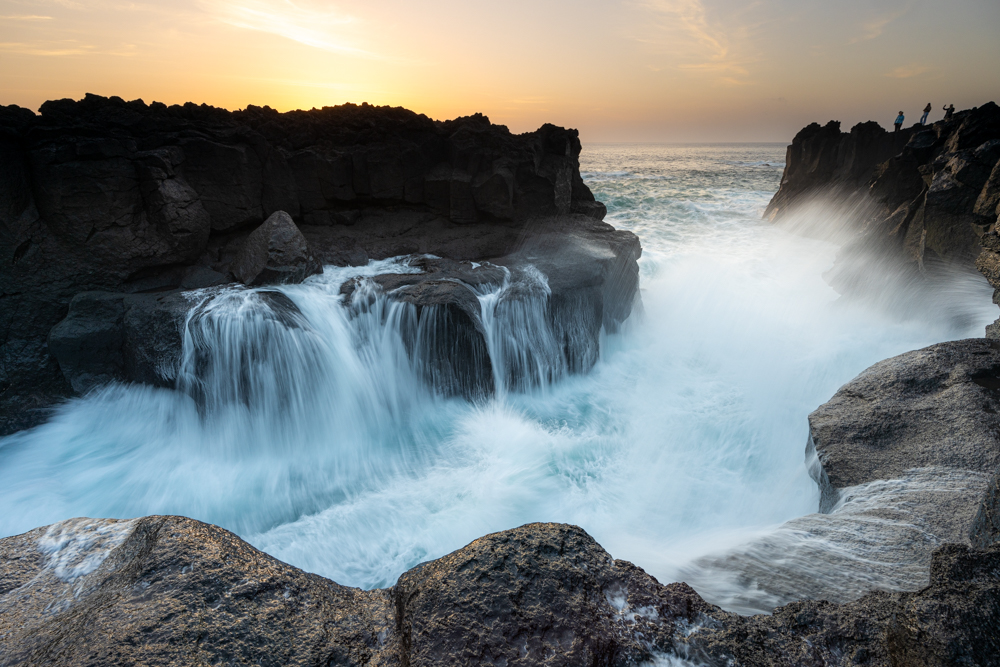The image showcases an awe-inspiring waterfall scene. At the very bottom, a gray rocky ledge serves as the foundation. From the right edge, a stream of water cascades down; the top section of this waterfall gleams in light blue hues. Adjacent to this, the water turns white and gradually fades in color towards the right. On the opposite side, another dark gray ledge with a rugged texture appears, adorned with light blue water streams trickling down. Beyond this ledge, a taller segment of the rock structure stands, its surface almost black. To the right, three silhouettes of people can be seen on another rocky outcrop, adding a sense of scale and wonder. In the center, an expanse of clear blue water opens up, providing a serene contrast to the dynamic waterfall. The sky above transitions from a gentle light purple at the horizon to a warm orange, eventually blending into a mix of pink and light purple higher up, completing the captivating scene.